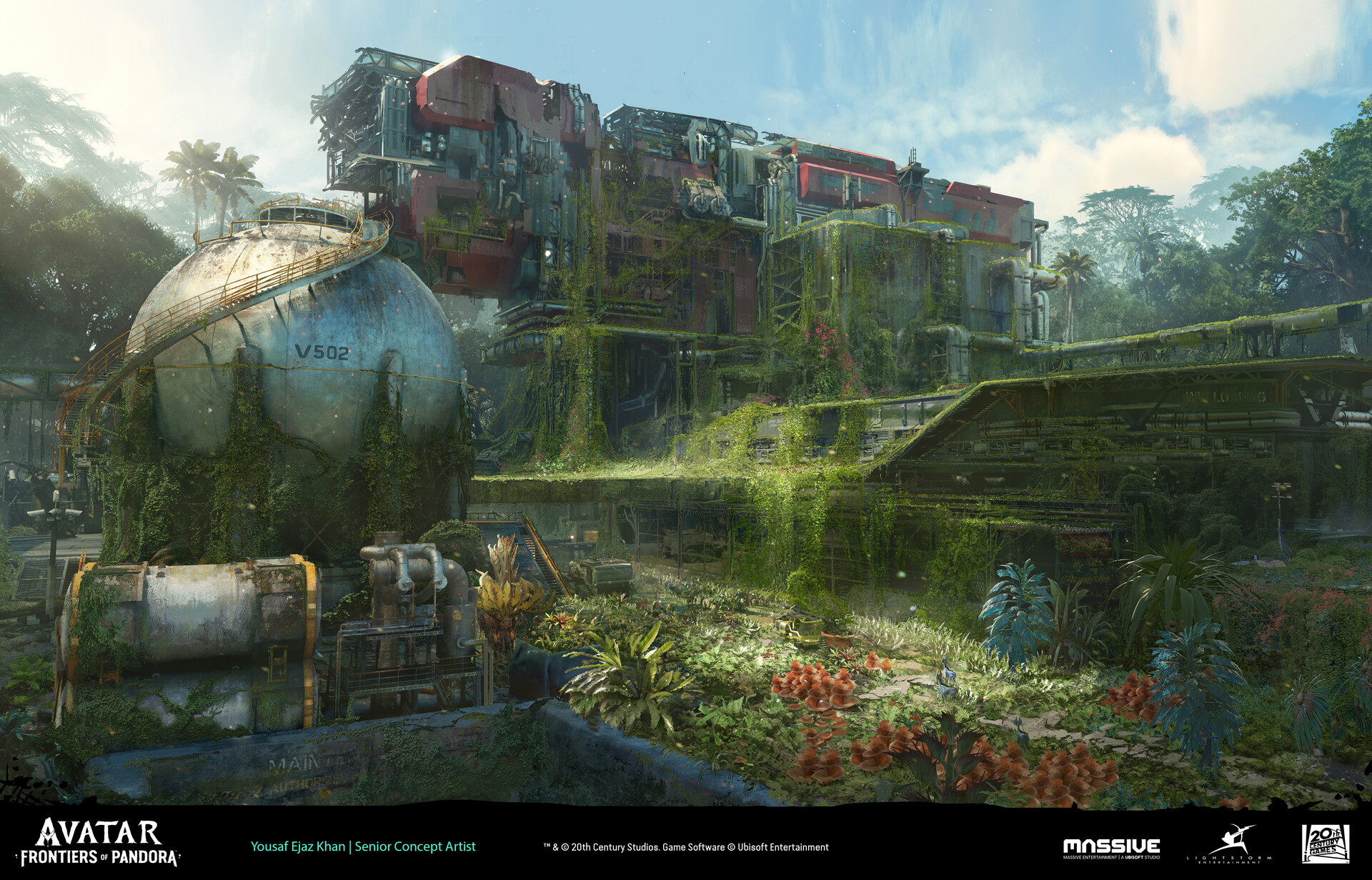This evocative image depicts a futuristic and abandoned living space, presumably within a fantasy game environment, specifically from "Avatar: Frontiers of Pandora." Conceptually crafted by Senior Conceptual Artist Yusuf Ijaz Khan from 20th Century Studios, the immersive scene is subtitled with the logo "Massive" and features a prominent 20th Century Studios logo in the bottom right corner.

The foreboding visual centers around a large spherical structure, possibly a chemical tank or water tower, engulfed in overgrowth. This colossal, steel-gray and white orb, draped in moss, complements an adjacent refinery plant that appears equally worn and overtaken by nature. The futuristic, red-painted refinery or base structure, elevated with a spiral staircase, is entangled with vines and foliage, suggesting years of abandonment.

The living area, enveloped in lush greenery, features an array of ferns, red flowers, and various plants thriving amidst the concrete and industrial remnants. The space leads ominously down into a pit, adding to the eerie atmosphere. The broader environment showcases a serene blue sky, scattered clouds, and towering trees, encapsulating an abandoned yet revitalizing juxtaposition of nature reclaiming a once-industrialized area.